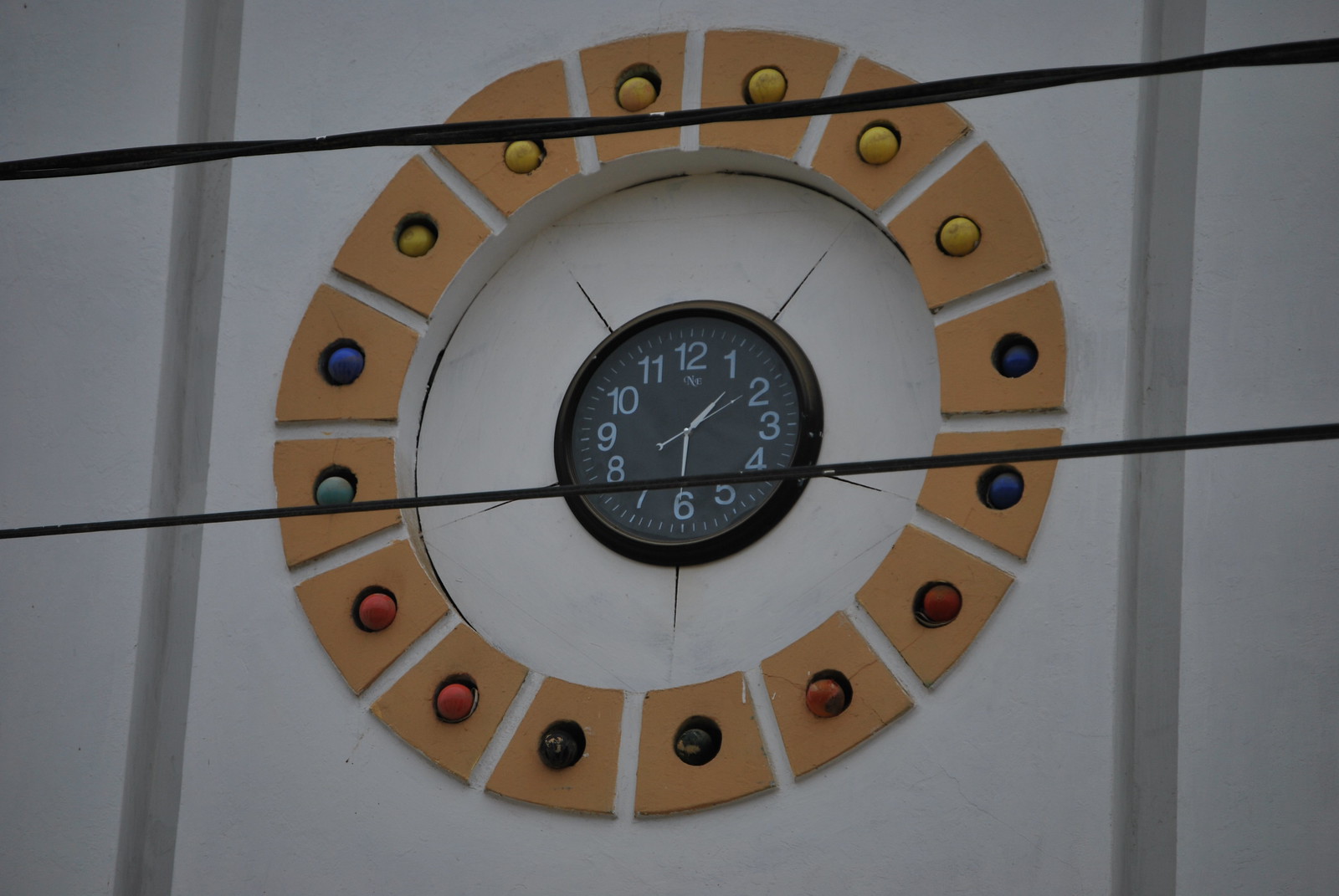The photograph captures a strikingly ornate clock mounting at what appears to be an amusement park or carnival setting. In the foreground, utility lines intersect the image, partially obscuring the view but adding an element of real-world clutter typical of such locations. The clock itself features a simple, dark analog dial with light bluish-green numerals and standard hour, minute, and second hands. It is encased in a dark bezel and prominently mounted at the center of a spherical structure.

This sphere, likely made of concrete or plaster, serves as a decorative frame for the clock. Surrounding the clockface is a beige or light brown circular area adorned with multi-colored bulbs, possibly chaser lights designed to create a dynamic and vibrant display at night. The background around the sphere consists of plaster or stucco with vertical gray lines set against an off-white surface, adding to the clock's visual prominence.

The setting exudes the chaotic charm and festive atmosphere of an amusement park or carnival. The colored bulbs, the slightly haphazard utility lines, and the vibrant, yet somewhat messy, surroundings all contribute to an environment bustling with activity and excitement. This clock undoubtedly serves as a whimsical and practical focal point for visitors, embodying the playful spirit of the venue.